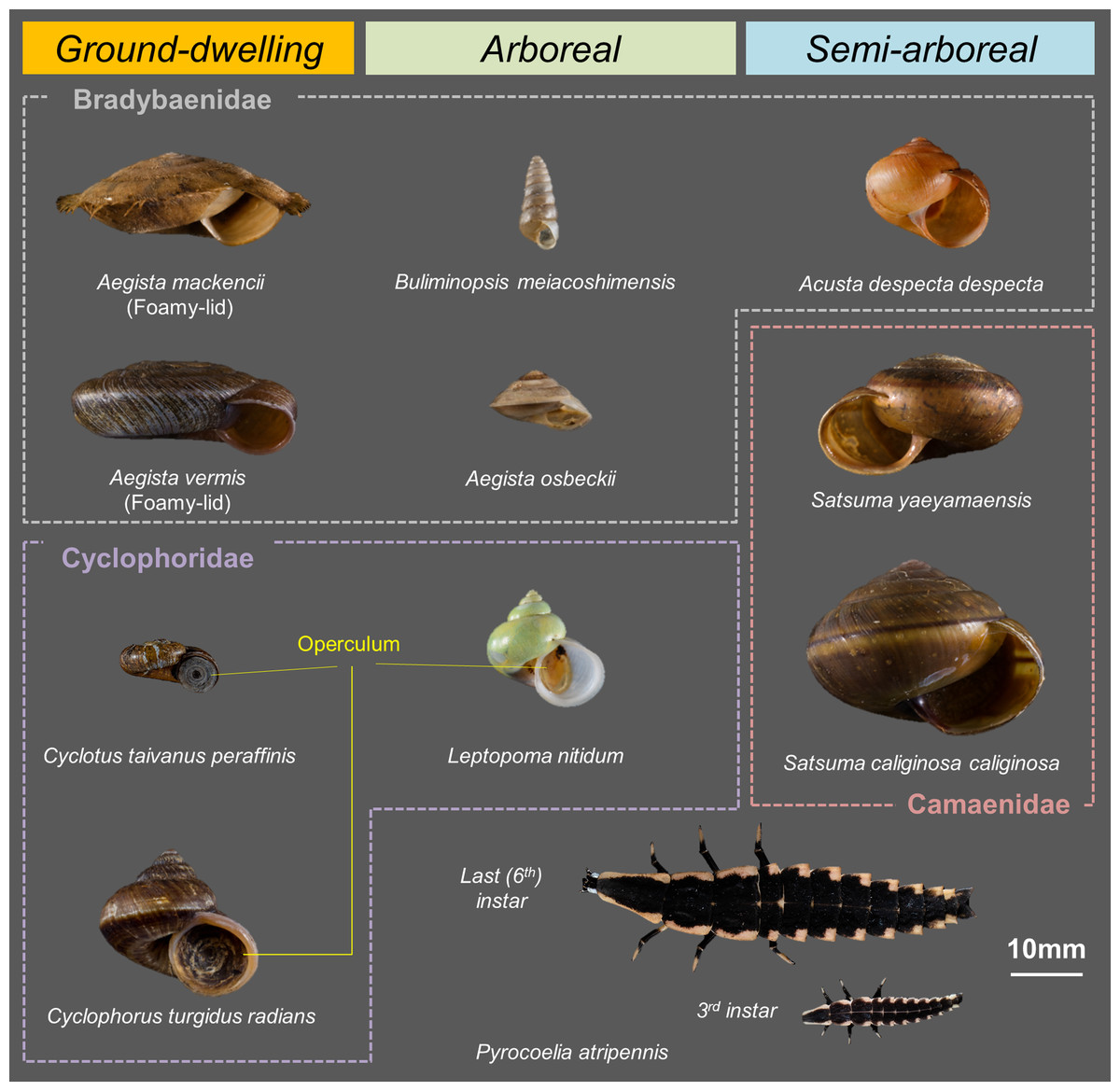This detailed infographic illustrates various types of shelled creatures categorized into three distinct types on a gray background. At the top, three thin, colored rectangles serve as headers for the categories: "Ground-dwelling" displayed in a yellow rectangle to the left, "Arboreal" in a green rectangle in the middle, and "Semi-arboreal" in a blue rectangle to the right. Below these headings are sections shaped like Tetris pieces, outlined with white and colored dotted lines. The ground-dwelling category features flat shells, the arboreal category includes tall, cone-shaped shells, and the semi-arboreal category presents a mix of cone-shaped and flat shells. 

Eleven scientific shells are displayed beneath these categories, each with a dotted-line outline leading to their labels, which detail their complex scientific names, such as "Buleminopsis miyakashimensis." Additionally, there's a segment at the bottom right showing an insect viewed from below, identified as "Pyrocoelia atripenis," resembling a larva with a long tail and six legs. Adjacent to this, a size guide features a large and small snail with a key indicating "10 mm." This comprehensive graphic effectively categorizes and labels different shell types and includes additional detailed biological illustrations for reference.